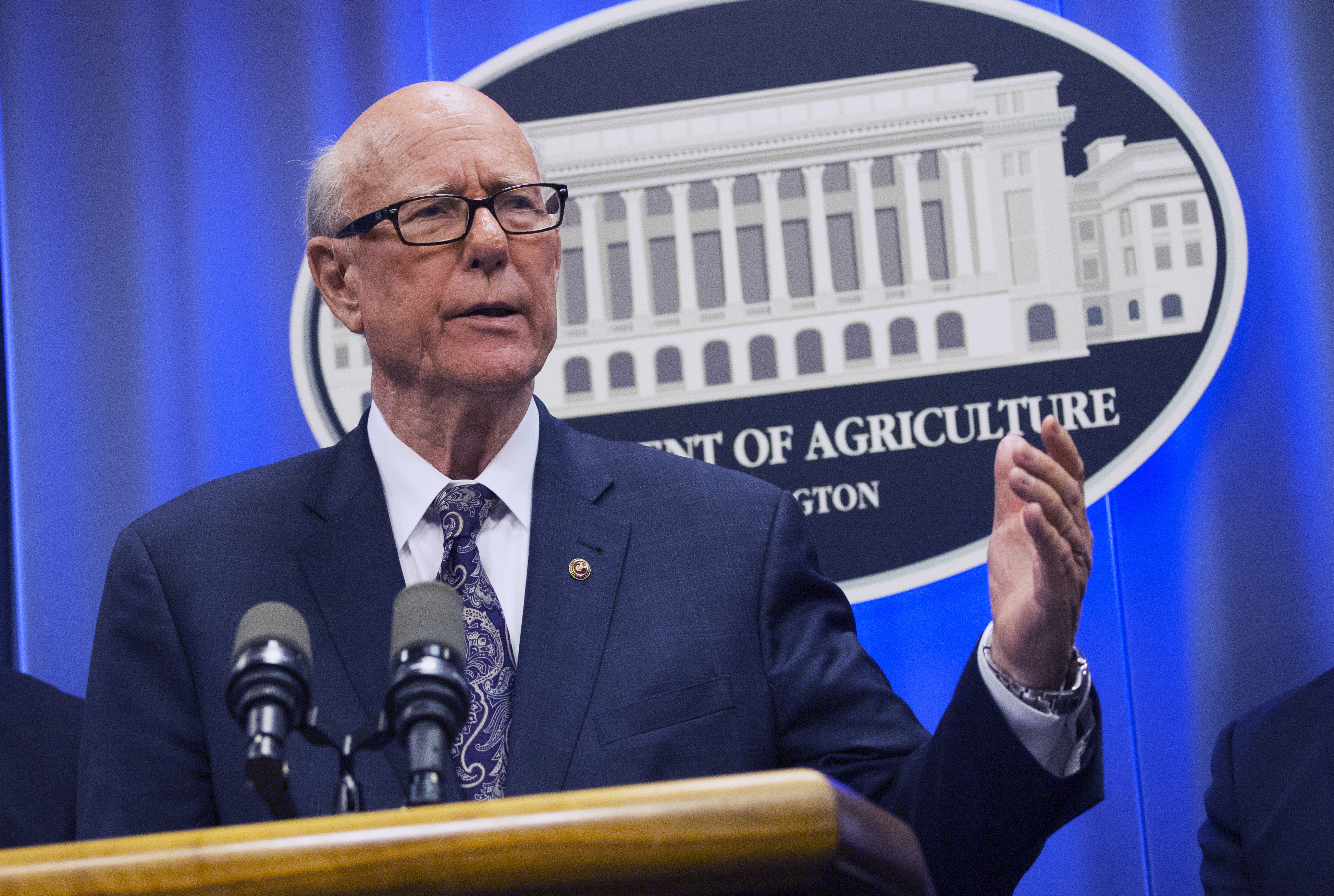The image features an elderly white man with gray hair and black glasses, standing at a brown, wooden podium equipped with two microphones. He is mid-speech, with one hand raised, dressed in a blue suit, vintage blue tie, and a white button-down shirt. The backdrop consists of a blue curtain with the partially visible emblem of the Department of Agriculture, featuring a depiction of a white building reminiscent of the White House. The man is the focal point, obscuring part of the inscription on the logo as he addresses the audience.